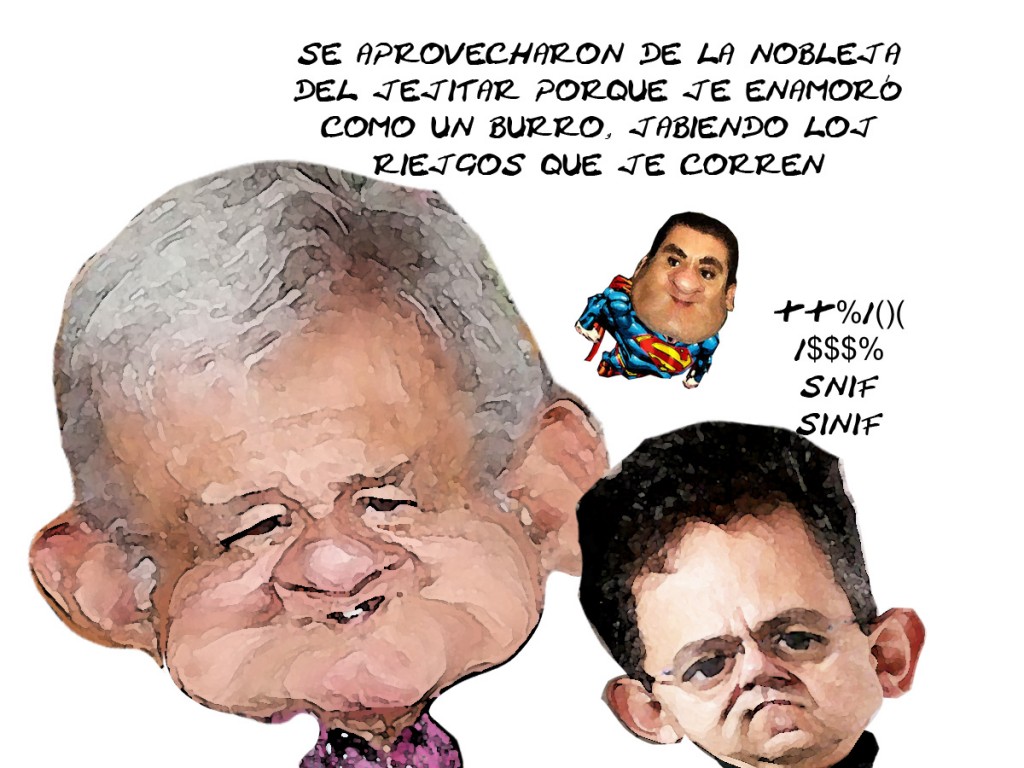The image depicts a detailed political cartoon featuring three exaggerated caricatures. The primary and largest figure on the left is a pale man with gray hair, large cheeks, oversized ears, and a broad smile, dressed in a pink shirt. Directly to his right is another significant face with black hair, large ears, and a frowning expression, contrasted with the smiling figure on the left. Above these two figures, there is a smaller caricature of a man with chubby cheeks, a very large nose, and black hair, dressed in a Superman costume, with his body disproportionately smaller than his head. The cartoon style is reminiscent of Snapchat filters, with exaggerated foreheads, cheeks, and other facial features. The image includes several lines of text in French, making a political statement that is not immediately clear. Additionally, there are various symbols, such as plus signs and parentheses, along with the phrase "sniff sniff" positioned above the third character, emphasizing the satirical and exaggerated nature of the drawing.